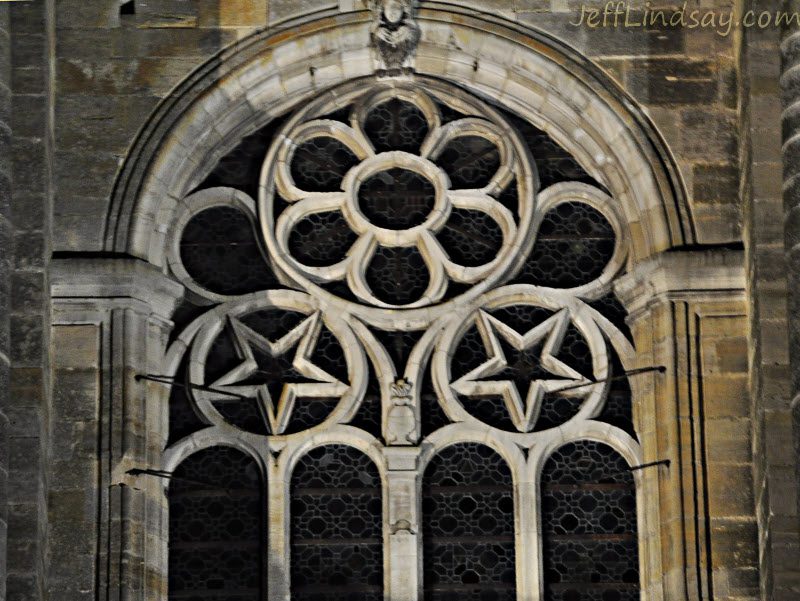This image features a close-up view of the façade of an old-style stone brick church, prominently showcasing a large, intricate stone archway. The archway, which forms the central element of the composition, is adorned with elaborate designs resembling flower petals, giving it a delicate and ornate appearance. Below this arch is a large circular motif with a smaller circle at its center, surrounded by petal-like stone patterns, creating a flower-like formation. Flanking the main circle are two smaller circles, each containing a star design, adding to the intricate stone decoration. Beneath these smaller circles are two narrower arched openings, featuring stained glass windows, their darkened patterns visible due to the lack of interior lighting. The stone walls surrounding the archway vary in color from dark gray to light beige. The right-hand side of the stonework is particularly illuminated by light, indicating the light source is from the left. The website JeffLindsay.com can be seen inscribed at the top right of the image.